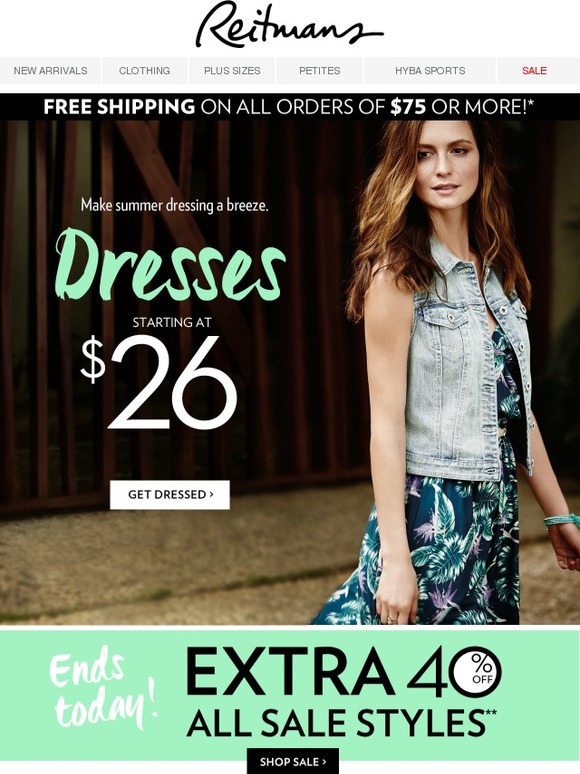**Detailed Description Caption:**

Three models are posing in a chic outdoor setting, standing in front of an intricately designed grey, gate-like backdrop which gives the impression of a wedding venue. The model on the left has vibrant red hair and is wearing a short-sleeved, open denim jacket layered over a blue dress adorned with floral patterns. The middle model is sporting a casual, sleeveless denim shirt paired stylishly with other summer attire. The model on the right wears a breezy mix summer dress that perfectly complements the relaxed atmosphere. 

The image promotes an ongoing sale by "Greatest New Arrivals" and "H-Y-B-S Sports," highlighting a special offer, where customers can enjoy pre-shipping on all orders of $75 or more. Dresses in the collection start at an affordable $26. A prominent green rectangle in the image reads, "Ends today! Extra 40% off all sale styles. Shop sale," urging viewers to take advantage of the significant discount. The website "www.larryweaver.com" is also featured for more information and shopping convenience.